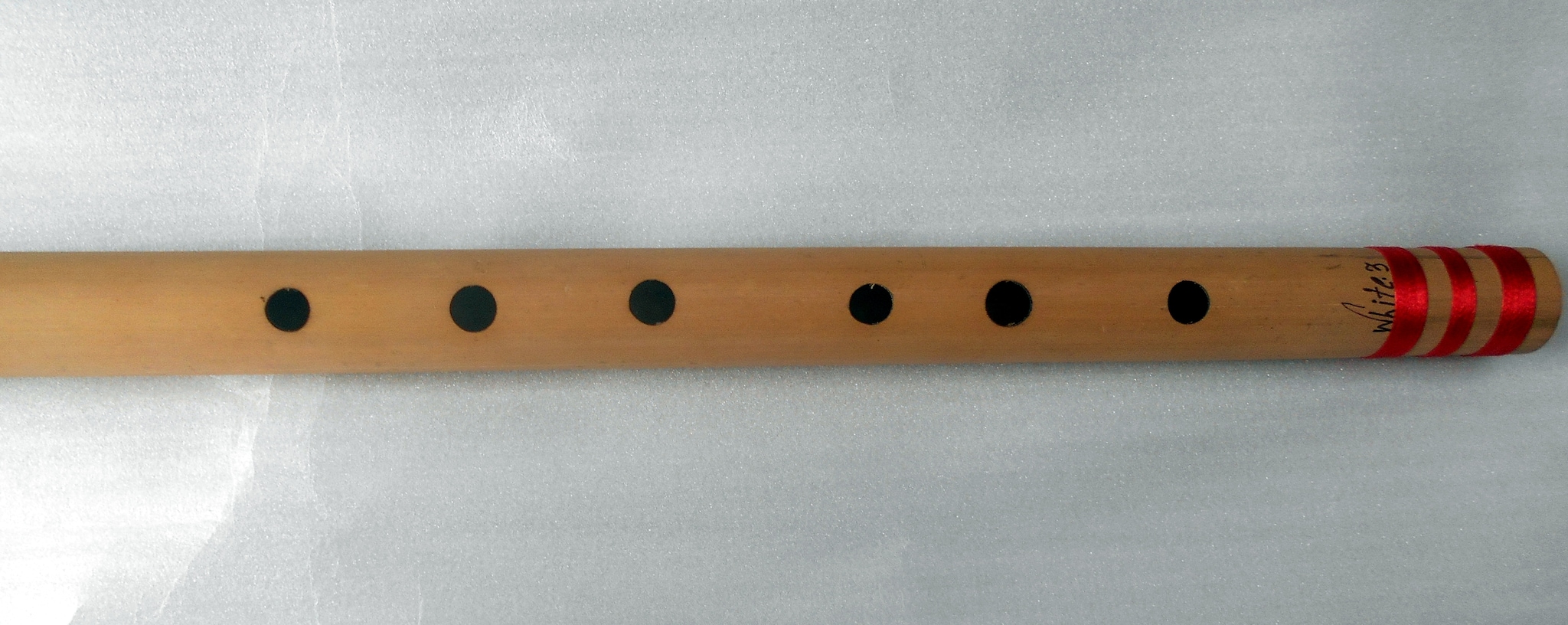This close-up image depicts a beige-brown cylindrical wind instrument, possibly of Asian origin. The instrument is displayed horizontally, with the mouthpiece on the right end, adorned with three shiny red rings. Six black dots, resembling finger holes, are aligned along the top surface of the instrument, although their spacing appears uneven, particularly towards the right side. The words "white 3" are handwritten on its surface. The background consists of a white cloth or paper, with lighting conditions creating a bright left side that gradually transitions to a grayer hue on the right.